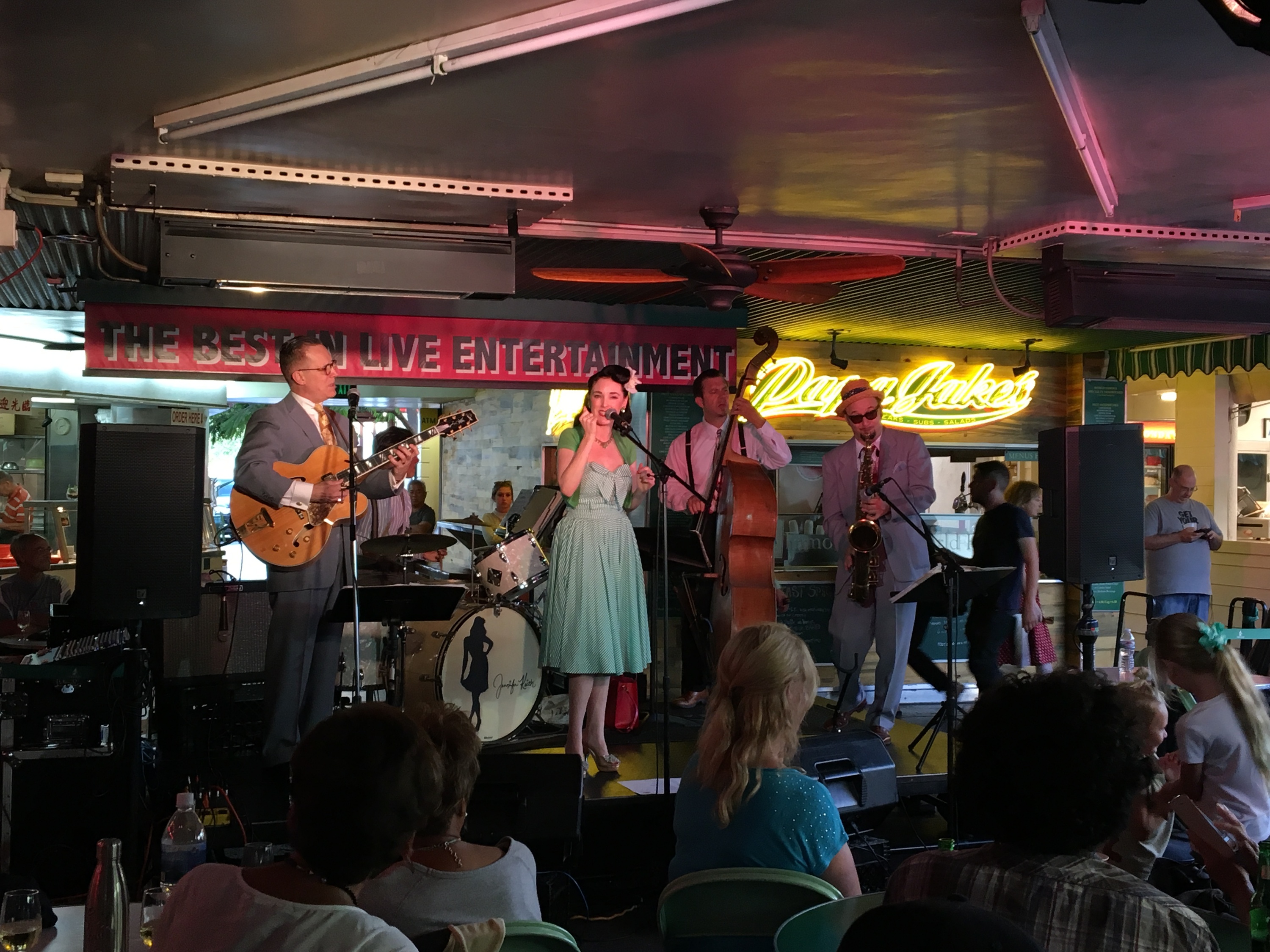The color photograph depicts a lively musical performance at a small venue, possibly a bar or restaurant, featuring a five-member band on a raised platform stage. The central performer, a woman with black hair adorned with a white flower on the right side, exudes a retro 1950s vibe, dressed in a vintage-style green A-line dress with a bow in the front, matching short-sleeved sweater, and high heels. She sings into a microphone on a stand. To her left, a man in a gray business suit with a tan tie and closely cropped dark hair, wearing glasses, plays an acoustic-electric guitar. Behind him, a drummer clad in suspenders and a button-up long-sleeve shirt is partially obscured, with the drum set featuring a picture of the same singing woman, alongside some script writing. 

To the right of the woman, a musician in a long-sleeve white shirt, black suspenders, and black pants skillfully plays a cello. Further right, another man, sporting a gray business suit, tan-colored hat, and sunglasses, passionately plays the saxophone. The backdrop of the stage features a prominent red banner proclaiming “The Best in Live Entertainment,” and additional lighting hangs overhead. An audience, seated in folding chairs, attentively watches the performance, adding to the intimate atmosphere of the scene, which resonates with a blend of vintage charm and contemporary execution.